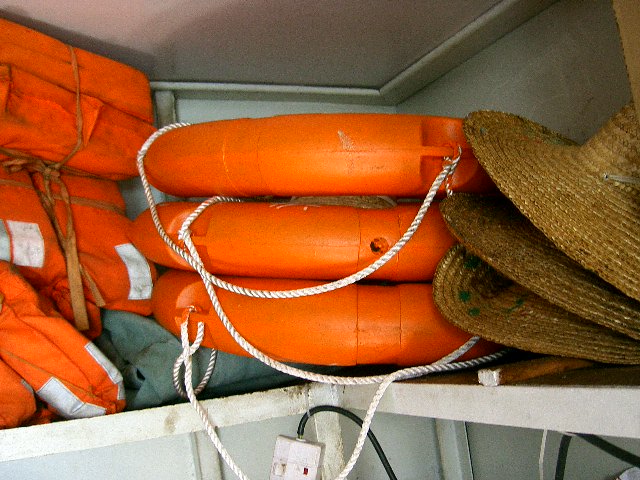The image depicts a small storage area, possibly on the front deck of a boat, filled with essential lifeguard and safety equipment. In the center of the wooden shelving are three bright orange rescue buoys, each equipped with white ropes and neatly stacked. On the left side, there are three orange life jackets, secured together with a brown, straw-like string. These life jackets are designed with straps for easy wear and secure fastening. To the right of the buoys, three wide-brimmed woven grass hats are stacked, offering sun protection with their large bills. Additionally, there is a folded blue item nestled between the life jackets and the buoys, and an extension cord extends from the wall, highlighting the practical and prepared nature of this storage space.